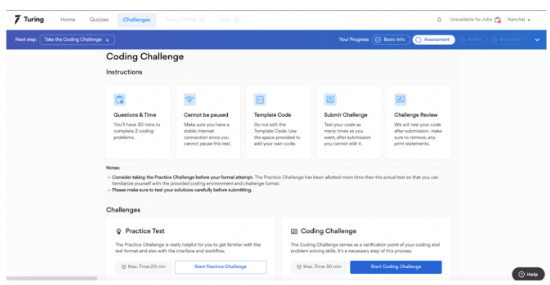The image is a detailed webpage layout. At the top is a white navigation bar with a logo resembling a 'T' or perhaps the number '7', followed by the word 'Turing'. To the right of this logo, the navigation menu includes 'Home', 'Guides', and 'Challenges'. In the top right corner, there are small icons including a bell and a dropdown menu.

Below the white navigation bar, there is a blue bar featuring additional navigational words with dropdown arrows. Underneath this blue bar, there is a section titled 'Coding Challenge Instructions'. This section contains five white boxes, each with a heading and a paragraph of text. Each box also has a small square icon in the top left corner. The headings for these boxes include 'Questions and Time', 'Cannot Be Paused', 'Template Guide', 'Submit Challenge', and 'Challenge Review'.

Following these boxes, there are additional paragraphs providing further instructions or information. Beneath these paragraphs, the section labeled 'Challenges' contains two large squares. The first square is titled 'Practice Test' and the second one is 'Coding Challenge'. Each of these squares includes descriptive text and a smaller square; notably, the 'Coding Challenge' square features a dark blue box, while a brown square at the bottom of the page is labeled 'Help'.